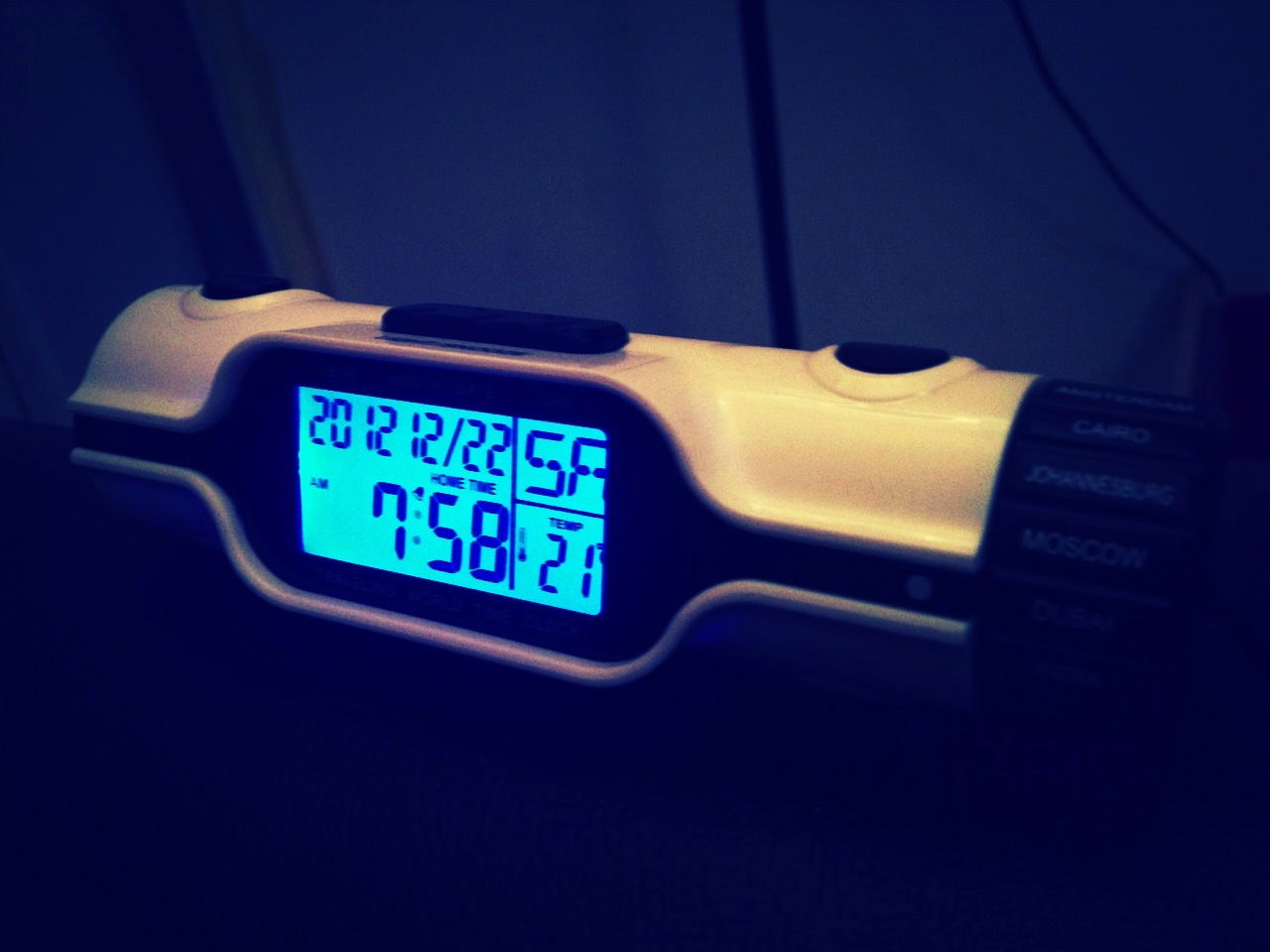This detailed caption highlights the comprehensive features and appearance of the clock based on the provided observations.

---

The photograph depicts a digital clock characterized by its sleek, tube-like shape with a silver and black color scheme. The clock is positioned lengthwise, lying on its side, and features a bright, glowing blue LCD screen with black numbers prominently displaying the time, 7:58 a.m. The digital interface combines several distinct elements: at the top, the date reads "2012/12/22," suggesting the clock's historical setting, while a black line divides the screen into sections. On the top right, the screen shows "SA" above a temperature reading of "21°C" (possibly Fahrenheit, though unconfirmed). Below, in larger font, the time "7:58 a.m." is labeled as "home time."

The clock is equipped with functional components, including black buttons and a dial situated to the right. This black dial allows users to switch between different city times such as Johannesburg, Cairo, and Moscow, indicating a world time feature. Additional buttons are located on the right and left sides of the device, and there’s a snooze button centrally placed on top. The rectangular screen layout protrudes slightly from the cylindrical body, enhancing its futuristic design. Overall, this clock is not only a timekeeper but also an innovative tool for tracking time across various global locations.